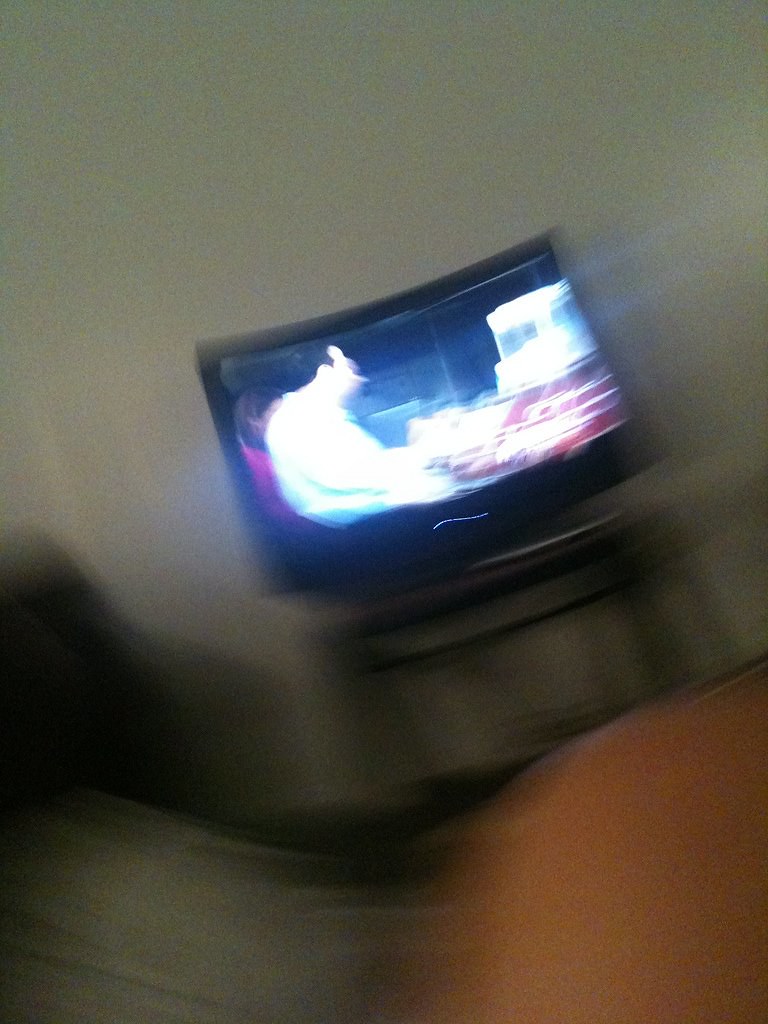A blurred portrait-style photograph features a small 40-inch television with a black frame, positioned against a grey wall. The TV, whose screen appears unfocused, rests on a compact brown table supported by slim black legs. In the lower right corner, the indistinct shoulder or arm of a person is visible, bathed in natural light. The entire image gives an impression of rapid motion, resulting in a significantly blurred and hazy appearance.